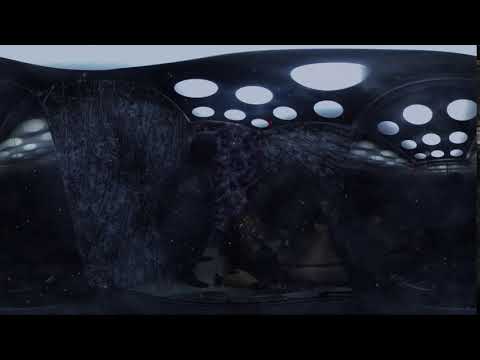The image depicts an otherworldly scene that could be interpreted as the inside of an alien cave or spaceship, or even an aquarium. The walls, resembling rock formations with intricate black veins, create a textured backdrop. There are several openings in the structure, including a small one and two larger ones. The ceiling is adorned with a variety of circular and oval lights. These lights range from small to large, arranged in patterns that appear random in some areas and more structured in others; one specific pattern above the smallest opening features three small, three medium, and three large lights lined up. The overall color palette is dominated by black and varying shades of gray, lending a mysterious ambiance. The ground appears to be composed of dirt or a grayish material. To the left, a hallway extends further into the scene, illuminated by additional lights. Amidst this alien landscape, a single small, pale yellow fish is visible, enhancing the surreal and enigmatic nature of the image.